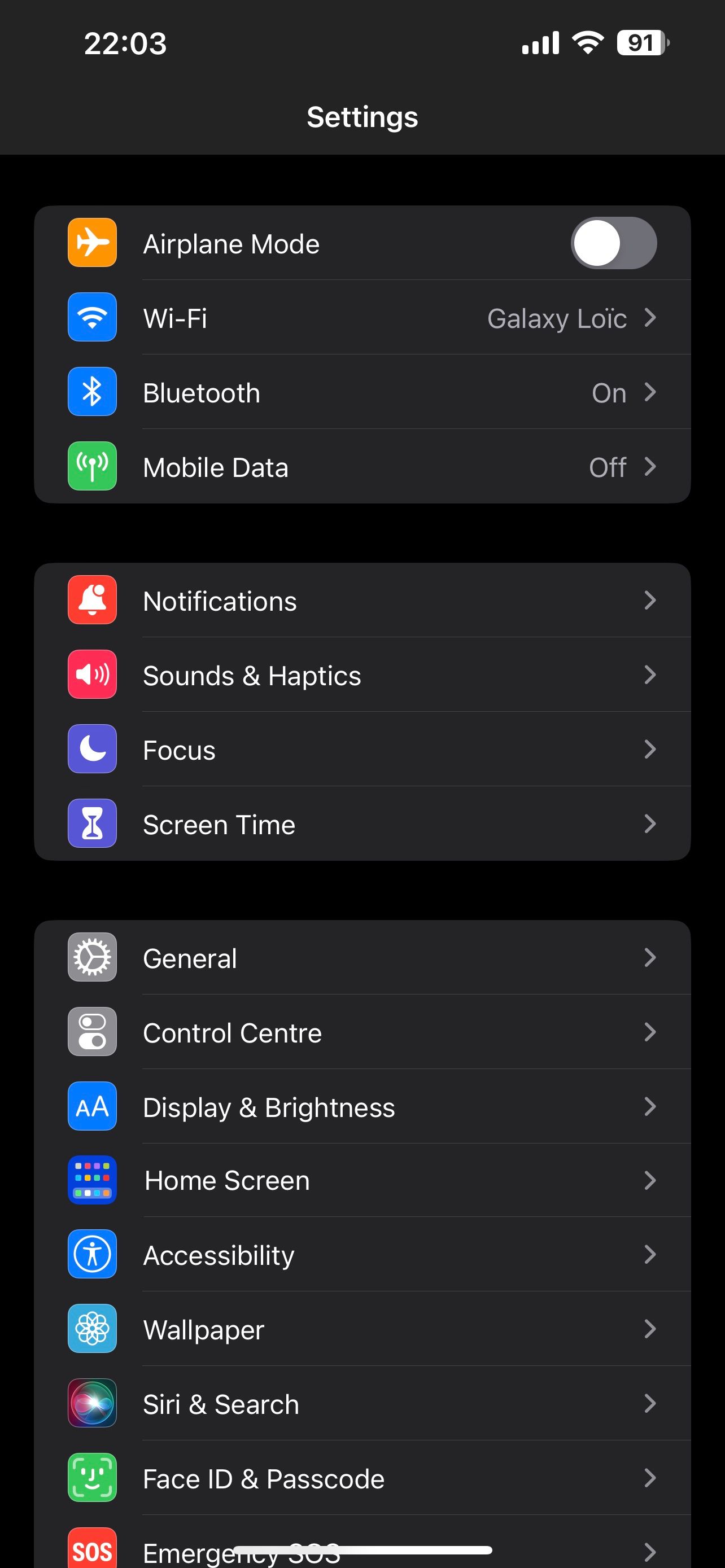This image is a detailed screenshot of a mobile device’s settings menu. At the very top left corner, the device displays the time as 22:03, with a cellular signal icon showing full bars. To the right, there is a wireless Wi-Fi signal icon and a battery icon displaying a charge level of 91%.

Centered below these icons is the heading "Settings," indicating the current section of the device. The settings menu is divided into several options indicated by icons and titles. 

- The first option features an orange airplane icon labeled "Airplane Mode," with a toggle showing it is deactivated.
- The second option has a blue Wi-Fi signal icon and the word "Wi-Fi," with "Galaxy Loic" indicated to the right, suggesting the device is connected to a network named "Galaxy Loic."
- Below this, a Bluetooth icon signifies that Bluetooth is turned on.
- A green mobile data icon and the words "Mobile Data" follow, with a dropdown indicating that mobile data is turned off.
- The next section has a red bell icon labeled "Notifications."
- Following that, a blue speaker icon is titled "Sound and Haptics."
- A purple moon icon with the title "Focus" comes next.
- Beneath this, a purple hourglass icon with "Screen Time" indicated.
- A gray gear symbol labeled "General" is the next option.
- Two gray button icons titled "Control Centre" (with the European spelling).
- Two capital A’s inside a blue square, representing "Display & Brightness."
- Multicolored dots labeled as "Home Screen."
- A person icon inside a blue square labeled "Accessibility."
- Additional options include "Wallpaper," "Siri & Search," "Face ID & Passcode," and "Emergency SOS," each with respective icons.

This comprehensive display captures a variety of settings options available on the mobile device.